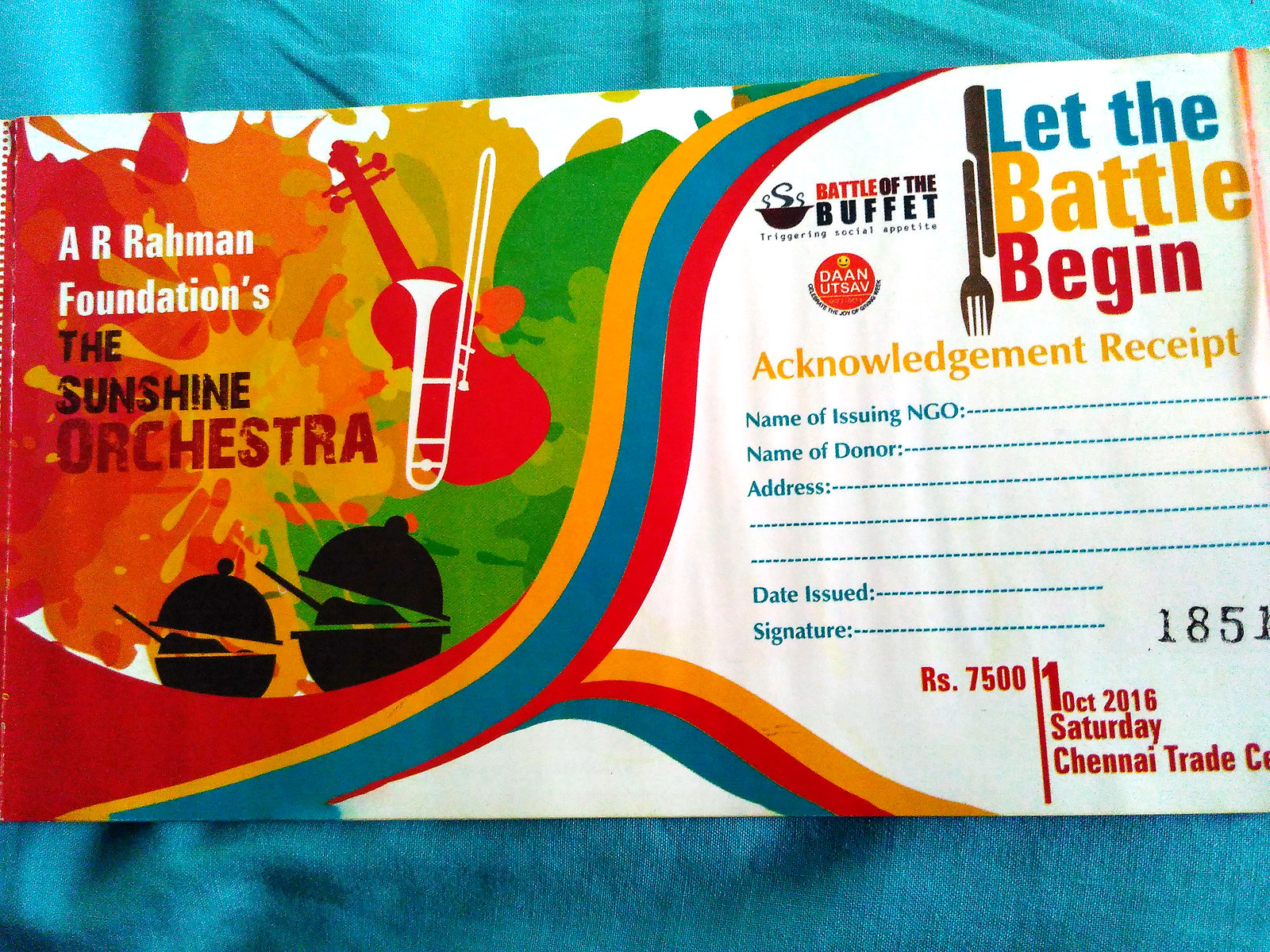The image is set against a teal blue, tablecloth-like background and features a colorful promotional or ticket form. On the left, it prominently displays "A.R. Rahman Foundations, the Sunshine Orchestra" accompanied by a digital illustration of musical instruments—a white trombone with its bell facing upward and a red violin tilted to the left. Surrounding these elements is a vibrant splash of colors including shades of red, orange, yellow, green, and white, adding a lively touch to the design. Below the orchestra information, there are illustrations of two black containers resembling barbecues or cooking vessels, encircled by stripes. On the right side of the form, bold text declares "Battle of the Buffet," followed by "Let the Battle Begin," with a fork and knife pointing downward beneath it. The section labeled "Acknowledgement Receipt" includes blank fields for details such as the "Name of Issuing NGO," "Name of Donor," "Address," "Date Issued," and "Signature." Moreover, the form specifies "Ticket Number 1851," with additional text mentioning "R.S. 7500, 10 October, Saturday, Chennai Trade Company," though parts of this information may vary or be cut off.